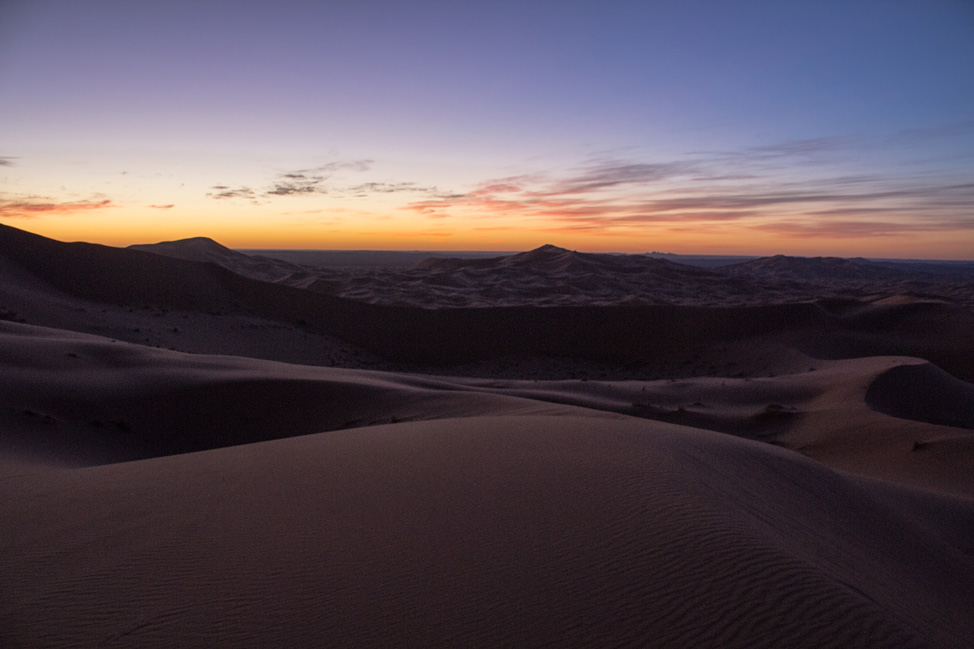This is a detailed landscape photograph capturing a desert scene at sunset. The overall lighting is dim, with the upper portion of the frame showcasing a sky transitioning through various shades of blue and purple, deepening towards the edges. Scattered, linear clouds stretch across the sky, while the horizon glows with a yellowish-orange hue from the recently set sun. The foreground features multiple darkly lit sand dunes, with intricate wind-blown patterns indicating a windswept environment. In the background, taller mountain ranges rise, with a distinct large dip or depression in the sand between the dunes and the mountains, creating a sense of depth and vastness in this tranquil yet dramatic desert landscape.